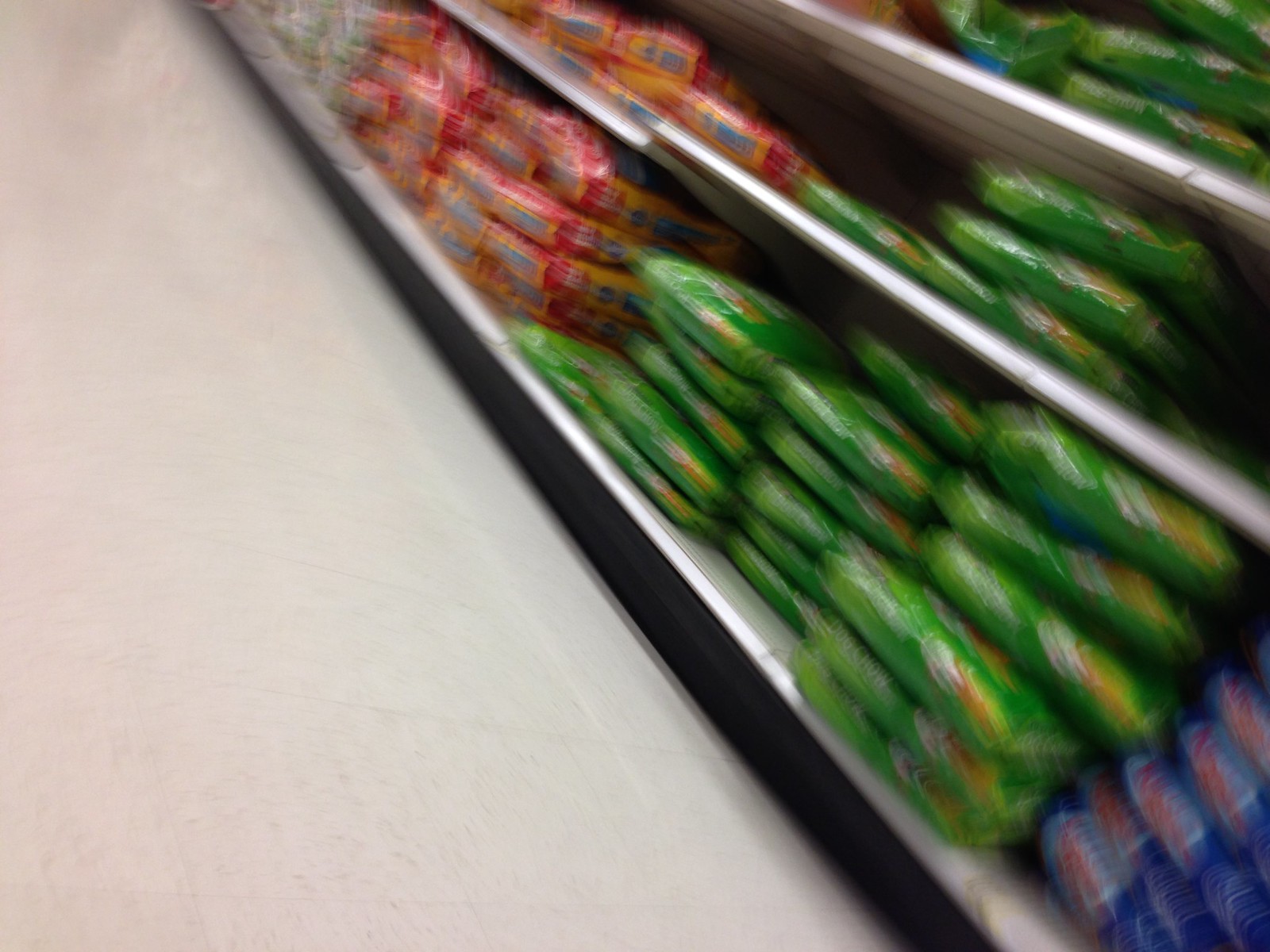The blurry image, likely taken inside a store while in motion, captures the lower rows of white shelving units running diagonally from the bottom right to the top left, almost dividing the rectangle-shaped picture in half. The flooring on the left side of the image is white linoleum, typical of store environments. The white shelves, topped with a black kickboard at the base, hold various colorful bags that could be pet food or garden supplies. The bottom shelf features a column of blue bags on the right, followed by three columns of green bags, two columns of red bags, and some white bags on the far left. This pattern repeats in diminishing quantities on the second and third shelves, with green bags being the most prevalent across all three levels.